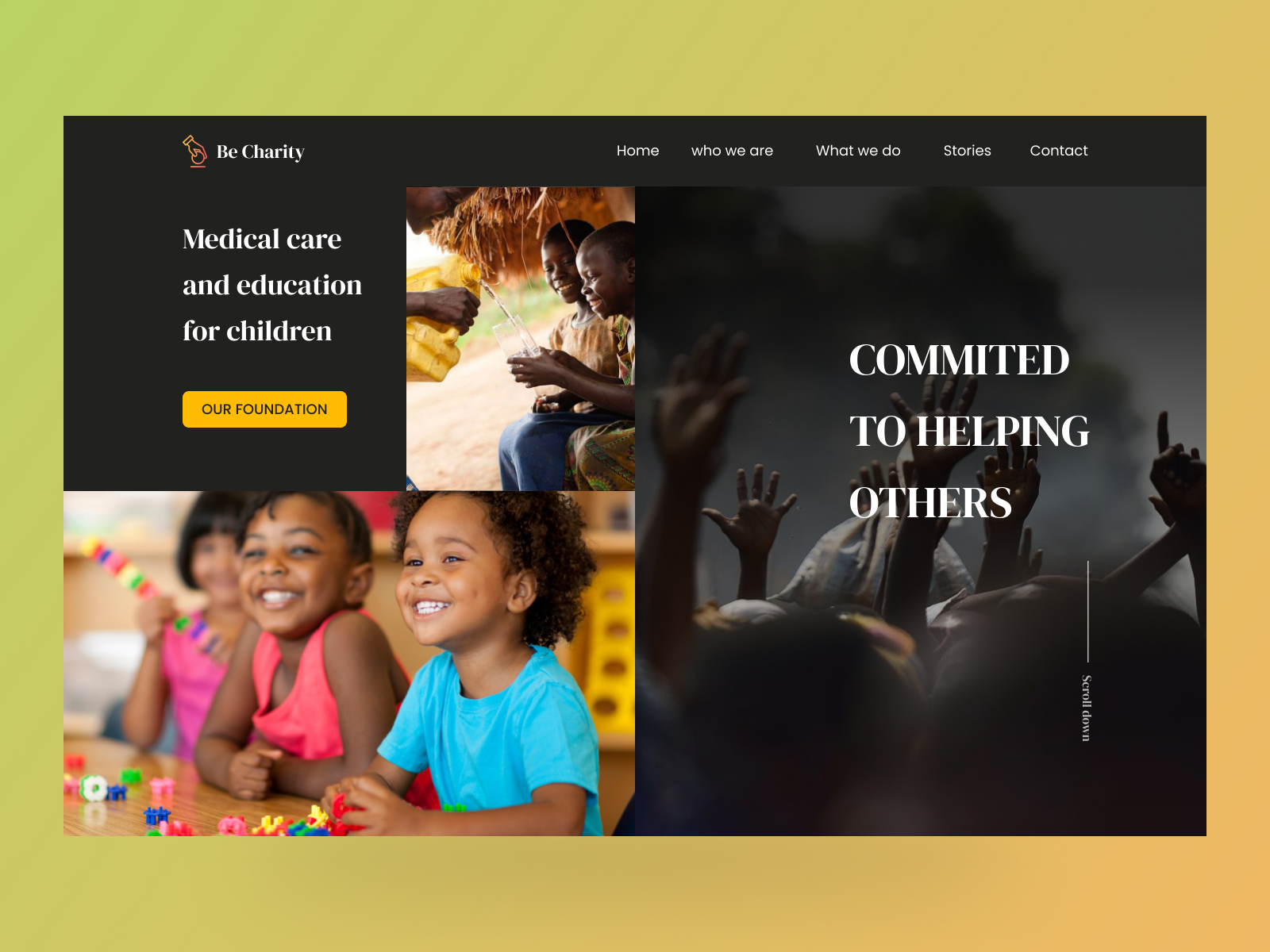The image features a screenshot that appears to be from a PowerPoint presentation slide, showcasing a detailed layout of a charity organization's website. The background of the slide has a gradient design, transitioning from green on the left to orange on the right. In the upper left corner, the website is branded with the text "Be Charity."

On the right side of the website layout, navigation buttons are listed, labeled as "Home," "Who We Are," "What We Do," "Stories," and "Contact." On the left side of the layout, prominent text reads "Medical Care and Education for Children," with a yellow button beneath it labeled "Our Foundation."

Adjacent to this text, there are two photographs. The first image shows two children receiving a glass of water from someone, emphasizing the theme of medical care. The second, lower photograph depicts three children in a classroom setting, engaging in play with building blocks, highlighting the emphasis on education.

Dominating the right side of the layout is a larger photograph of people's hands raised in the air, overlaid with the text "Committed to Helping Others." The photo includes a credit attributing the photographer.